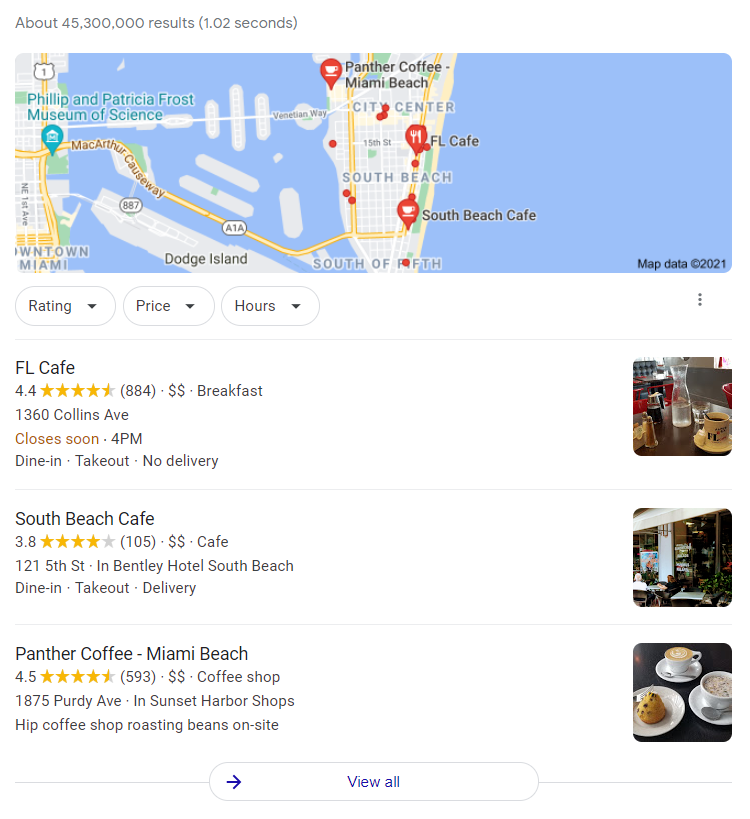This detailed caption describes a screenshot of search results for cafes and coffee shops in the South Beach area of Florida. The top portion of the screenshot features a map with several red pins indicating the locations of various dining spots. Two pins display a coffee cup icon, and one pin shows a fork and knife, symbolizing cafes and restaurants. 

Below the map, specific search results are listed:

1. **FL Cafe**:
   - Rating: 4.4 stars out of 5
   - Description: Serves breakfast and closes at 4 p.m.
   - Address: 1360 Collins Avenue
   - Accompanying Image: Picture of the restaurant's interior or a table with food and coffee items.

2. **South Beach Cafe**:
   - Rating: 3.8 stars out of 5
   - Description: Offers dine-in, take-out, or delivery services.
   
3. **Panther Coffee - Miami Beach**:
   - Rating: 4.5 stars out of 5
   - Description: A hip coffee shop known for roasting beans on-site.

Each result is accompanied by an image showcasing either the interior of the establishment or a table set with food and coffee.